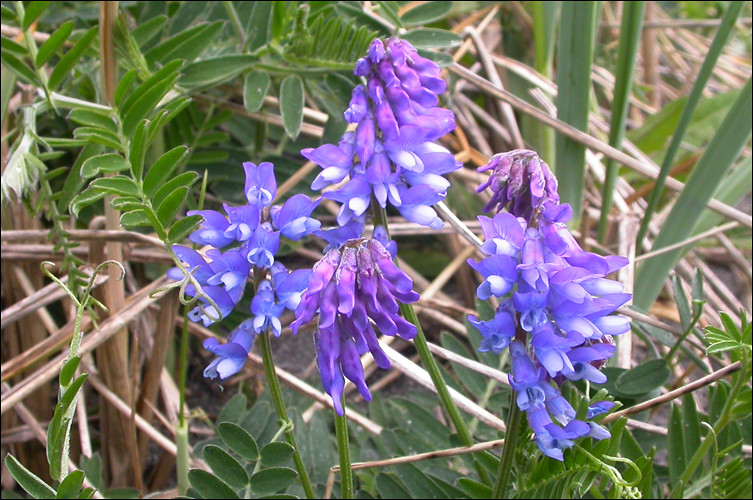This close-up photograph, taken outdoors, captures a cluster of delicate purple flowers with white-tipped petals. Each flower exhibits long, thin, and slightly oblong petals that do not fully open, forming distinct, yet not fully bloomed buds. The image showcases four to five of these intricate blossoms, each held by slender green stems adorned with oval-shaped leaves. The flowers are set against a backdrop of dense vegetation, including tall pieces of grass, vine-like plants, and thin, tan branches, which all contribute to a lush and natural setting. Despite the close-up focus on the flowers, the presence of various green plants and branches both in the foreground and background suggest a rich and thriving environment.